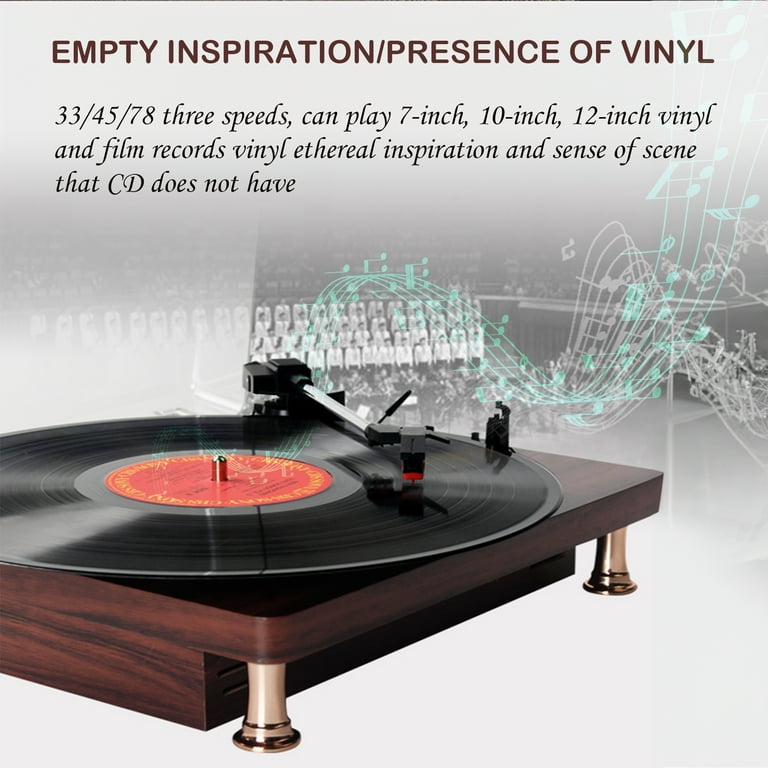This is a detailed color photograph of a vintage turntable, showcasing a sophisticated stereo record player set on a rectangular wooden platform with elegant brass and white legs. Dominating the player's surface is a large black vinyl record with a distinctive center label in red adorned with yellow and black text. The tonearm is positioned on the record, indicating that it is in the midst of playing.

The backdrop of the image is a gray hue punctuated by whimsical green music graphs and semitransparent imagery of a black-and-white choir or orchestra, giving a sense of musical history and ethereal inspiration. At the top of the image, bold text in brown and black italicized lettering reads "Empty Inspiration / Presence of Vinyl" followed by specifics, "33 / 45 / 78, three speeds, can play 7 inch, 10 inch, 12 inch vinyl and film records, vinyl ethereal inspiration and sense of scene that CD does not have." This textual overlay emphasizes the unique auditory experience and nostalgic quality that vinyl records provide, contrasting them with the more sterile feel of CDs.